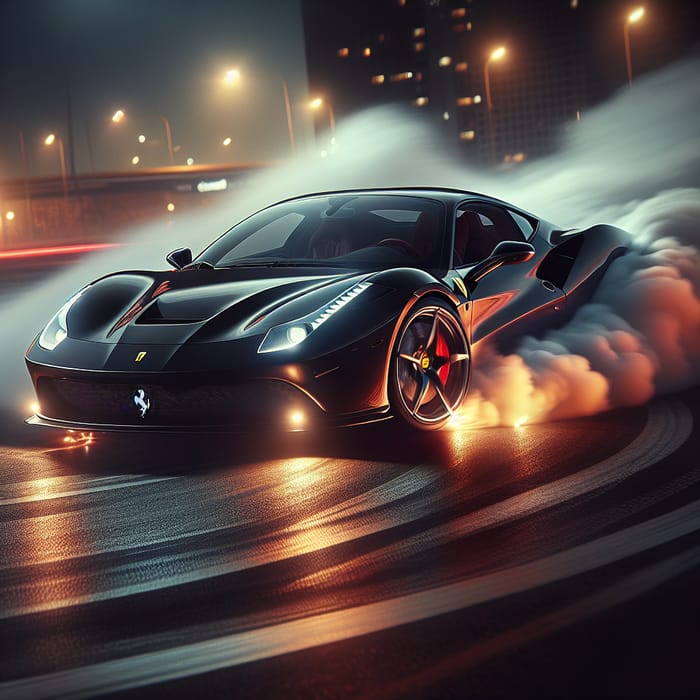The image depicts a sleek black sports car, possibly a Ferrari, careening through a cityscape at night. The 3D illustration captures the car mid-drift, with dense, swirling smoke billowing from its tires, emphasizing its high speed and aggressive maneuvering. The scene is rendered in a horizontal layout, and the backdrop features blurred city lights and street lamps, accentuating the car's rapid motion. The vehicle’s front end hints at a Ferrari with a vague yellow emblem resembling the iconic prancing horse, though inconsistencies, like an additional emblem below, suggest the image might be AI-generated. The interior of the car appears empty, missing a driver, which adds to the surreal quality of the portrayal.